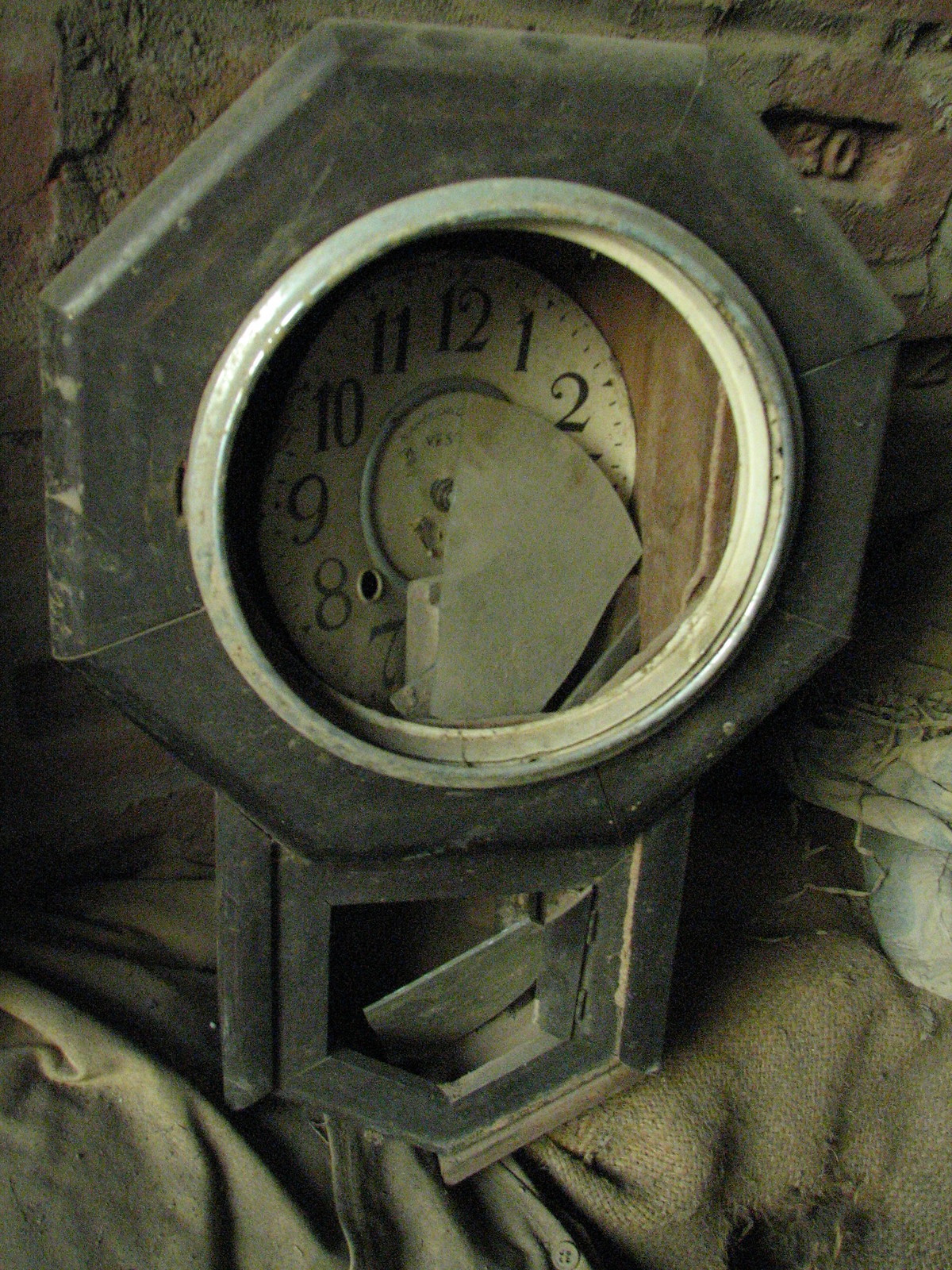The photograph captures a vintage Dakota grandfather clock, a compact model no taller than two feet, designed to hang on a wall. Distinct from the usual brown wood, this clock is finished in black. Its condition is notably deteriorated: the striker is non-functional, the glass door protecting the pendulum is shattered, and the glass over the clock face is similarly broken, with a shard resting against the dial. The clock hands are missing or obscured, all cloaked in a heavy layer of dust and grime. The clock is propped against a rustic brick wall, atop a piece of canvas. Attached to the wall is an old metal weight, estimated to be 20 or 30 pounds. This adds to the scene's atmosphere of neglect and faded grandeur.